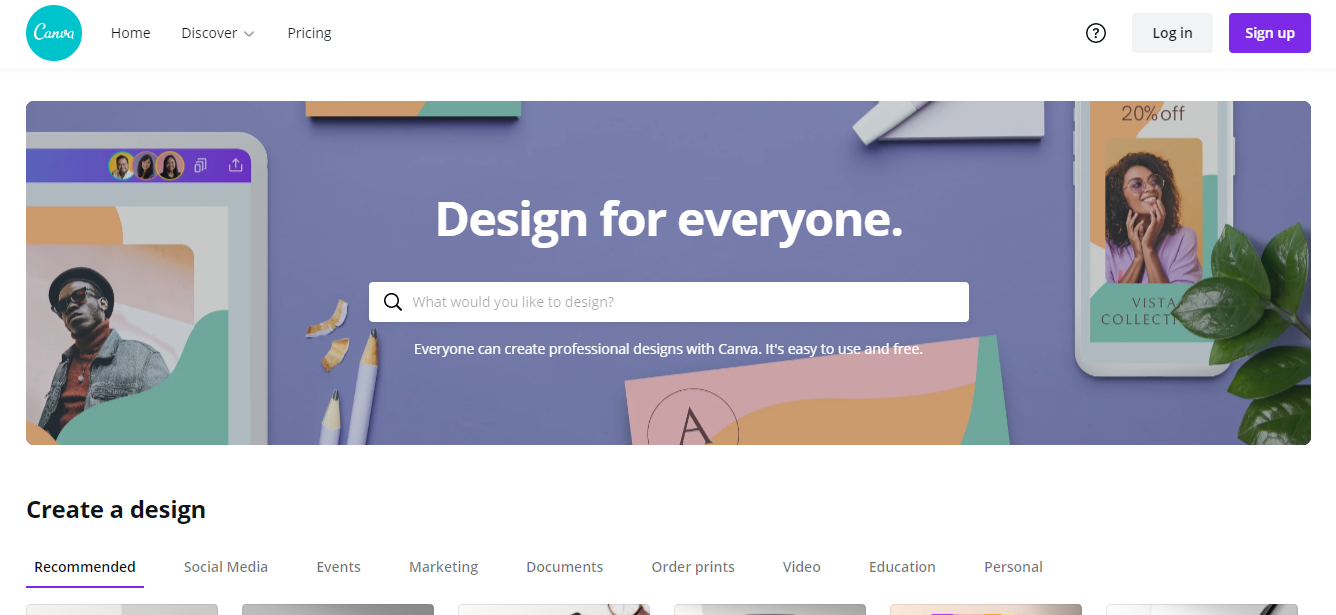This photograph captures the home page of the Canva website, prominently showcasing its user-friendly design. In the upper left-hand corner, the recognizable Canva logo—a circle containing the word "Canva"—is visible. The navigation bar at the top offers several options: "Home," "Discover" (which includes a drop-down menu), and "Pricing." On the far left, there are icons for help (represented by a question mark), login, and sign-up.

The main section of the page is dominated by a striking periwinkle blue rectangle. Within this rectangle, two photos are prominently displayed—one of a smartphone and the other of an iPad. Bold white text spells out, "Design for everyone," emphasizing Canva's inclusive design philosophy. A white search bar positioned below this slogan asks, "What would you like to design?" Just beneath, it reassures users with the message, "Everyone can create professional designs with Canva. It’s easy to use and free."

Additional graphical elements on this page include colorful pencils and pads of paper. Below the main call to action "Create a design," users are presented with a range of categories to choose from: "Recommended," "Social Media," "Events," "Marketing," "Documents," "Order Prints," "Video," "Education," and "Personal". To the far right of the image, part of a green, shiny-leaved plant is visible, adding a touch of nature to the otherwise digital scene.